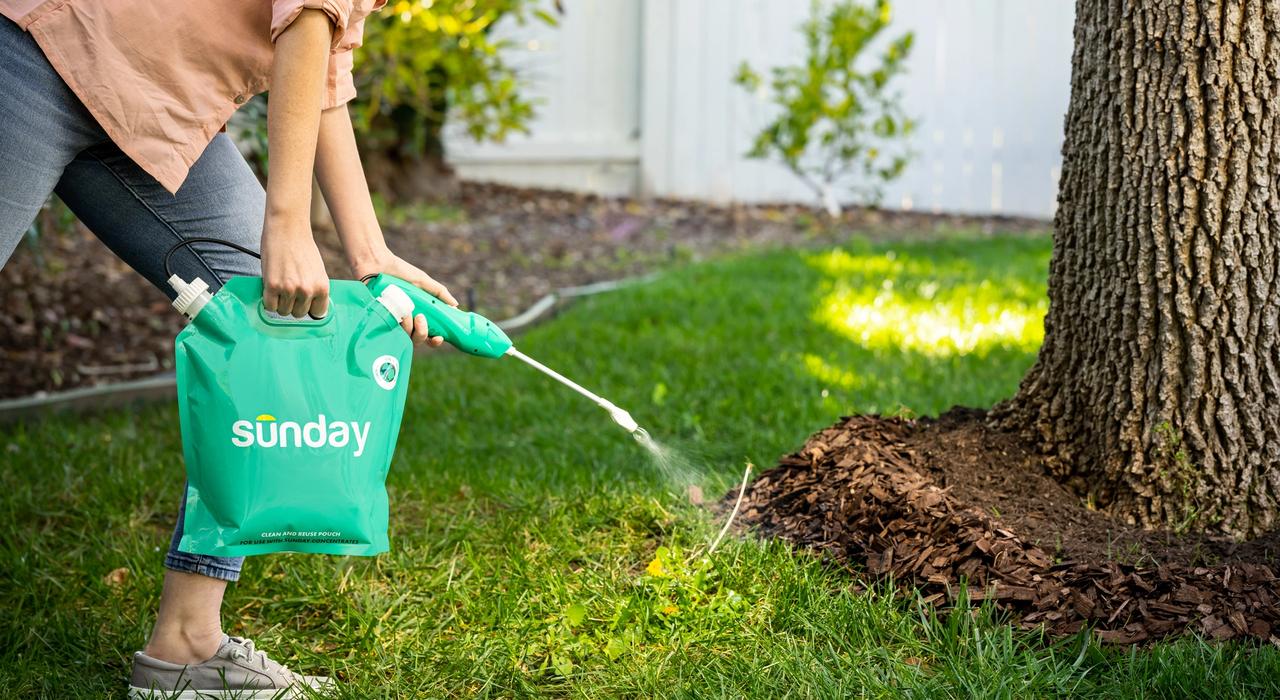This detailed image captures a moment of yard work, focusing on an individual, whose upper half is cropped out, engaged in weed control. The person, dressed in a light peach short-sleeve shirt, blue jeans cropped above the ankle, gray sneakers, and no socks, is positioned on the left side of the image. They are holding a mint green pouch with a spray nozzle, marked with the white logo "Sunday" and a small yellow sun above the "U", and are actively spraying weeds with visible droplets. The surroundings include a close-up view of green grass, partially blurred young saplings in the background, and a white wooden fence that's cut off at the top. The right-hand side of the photo features a tree trunk with distinctive rough bark, surrounded by brown mulch and soil. The image is bathed in daylight, illustrating the vibrant greenery and the detailed landscape, including the bordering mulch partition and the encroaching branches from nearby bushes.